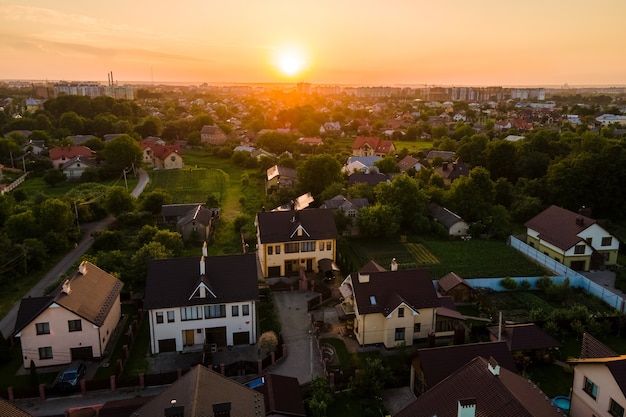This vibrant color photograph captures an aerial view of a suburban neighborhood at either sunrise or sunset. The center-left of the image showcases a glowing golden sun, casting warm hues and elongated shadows across a sprawling valley dotted with trees and greenery. The sun's light paints the clouds in stunning shades of orange and pink, adding to the image's serene and inviting atmosphere. 

In the sharper-focused foreground, we see an array of large A-frame houses with dark brown roofs, some appearing to be stucco, surrounded by green lawns and scattered trees. Roads weave through the neighborhood, guiding the eye towards the background where the scene transitions into a cityscape with larger buildings and possibly factories, evidenced by chimneys.

The horizon and distant buildings are in soft focus, creating a dreamy backdrop that contrasts beautifully with the detailed foreground. This image provides a rich and detailed view of a housing estate, blending the tranquility of suburban living with the distant hum of city life.